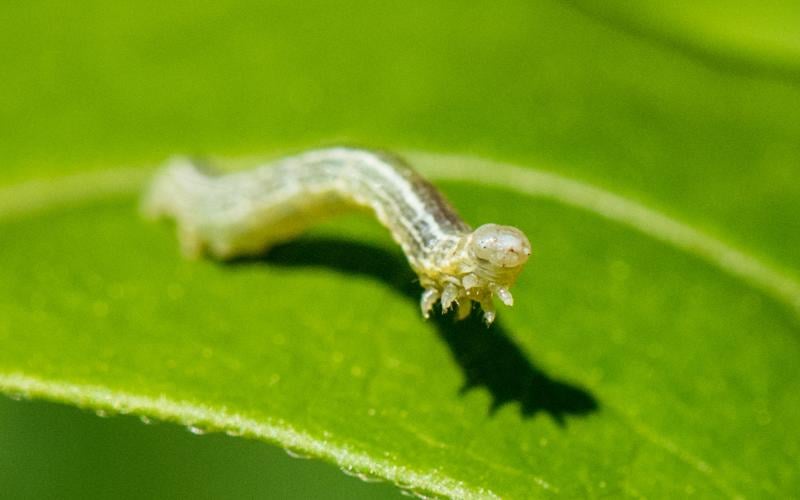The image is a horizontal, rectangular close-up of a caterpillar-like insect's face. The caterpillar's face is in focus, showing tiny black dots and six small, tentacle-like arms. Its tan-colored body has alternating dark brown and white stripes that become a lighter shade towards the tail, which blurs out as it extends backward. The background is a solid green leaf, featuring lighter green veins and some fibers, with a vivid lime green hue and yellow lines adding texture. The caterpillar is positioned diagonally from the mid-left to the center of the image, appearing to move forward with its front part raised, akin to an inchworm's motion. A shadow of the insect is also visible on the leaf.